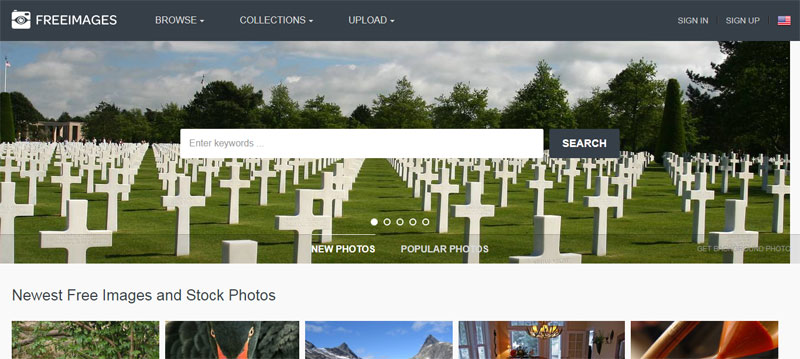The webpage titled "Free Images" features a clean design with a slightly navy background at the top, where the site name is prominently displayed. Navigation tabs including "Free Images," "Browse," "Collections," and "Upload" are aligned horizontally at the top. On the top right corner, users will find buttons for "Sign In" and "Sign Up," with the language set to United States English. 

In the center of the page, there is a navy-colored search bar labeled "Enter Keywords" for easy searching of images. Below this, sections labeled "New Photos" and "Popular Photos" are present.

The background image is a serene picture of a cemetery with nine white crosses in the foreground and lush green trees against a blue sky with grey and white clouds. There are navigation dots indicating slideshow functionality, with the first dot highlighted in white, and three unhighlighted white dots, suggesting the presence of more images to explore.

At the bottom left, labels read "Newest Free Images" and "Top Photos," featuring five slightly cut-off images. The central image showcases a vivid blue sky with grey mountains. To the left, there is an image of green plants with brown branches, followed by a black bed with gold eyes as accents.